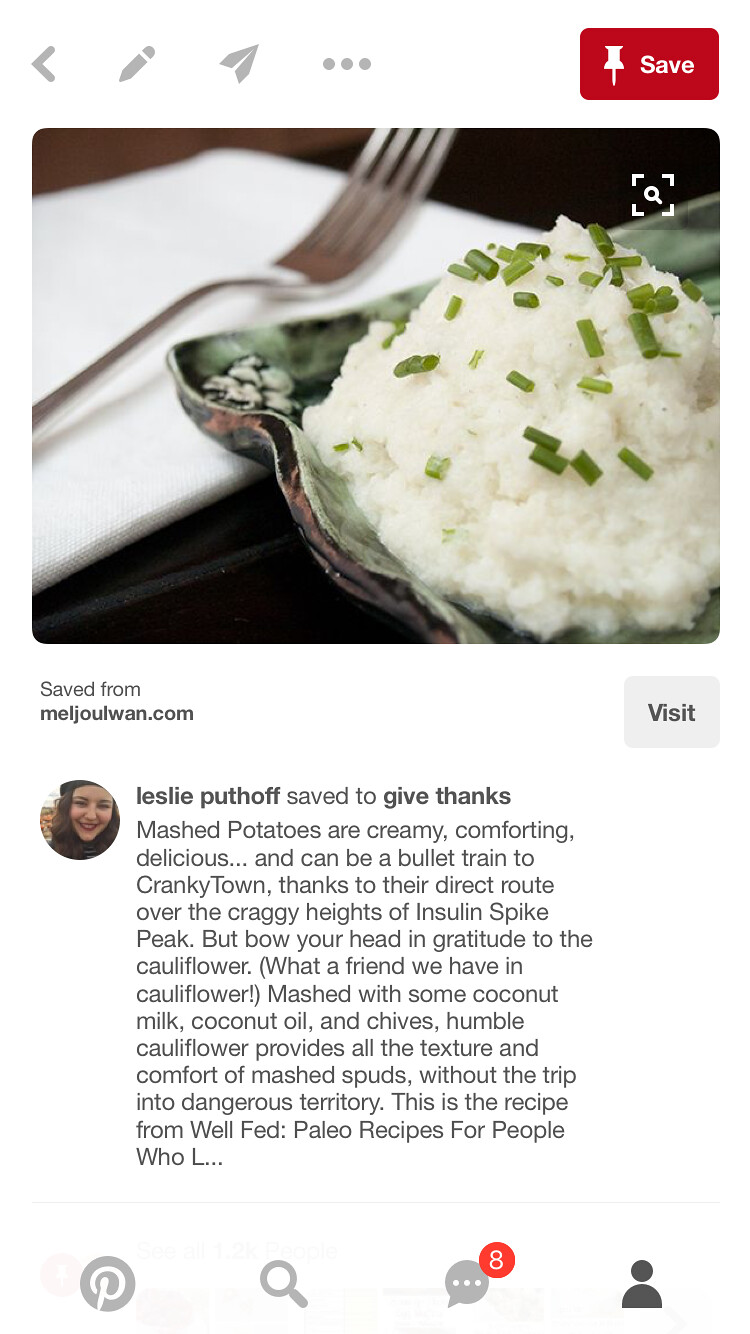This is a screenshot of a Pinterest post from Leslie Puthoff, originating from MelGillJuan.com. The interface displays a prominent red save button and a series of gray icons including an arrow, pencil, paper airplane, and ellipsis at the top. Below these are different icons for Pinterest actions, including a magnifying glass and messaging with an indicator showing eight messages. The central image features a mouth-watering dish of creamy mashed potatoes, garnished with green onions on a silver plate, with a blurred fork in the background. This image is accompanied by detailed text extolling the virtues of using cauliflower as a healthier alternative to traditional mashed potatoes. The description notes that mashed potatoes are delicious but can lead to insulin spikes, whereas cauliflower mashed with coconut milk, coconut oil, and chives offers similar texture and comfort without the health risks. The text cuts off with a mention of this being a recipe from "Well Fed Paleo Recipes for People."